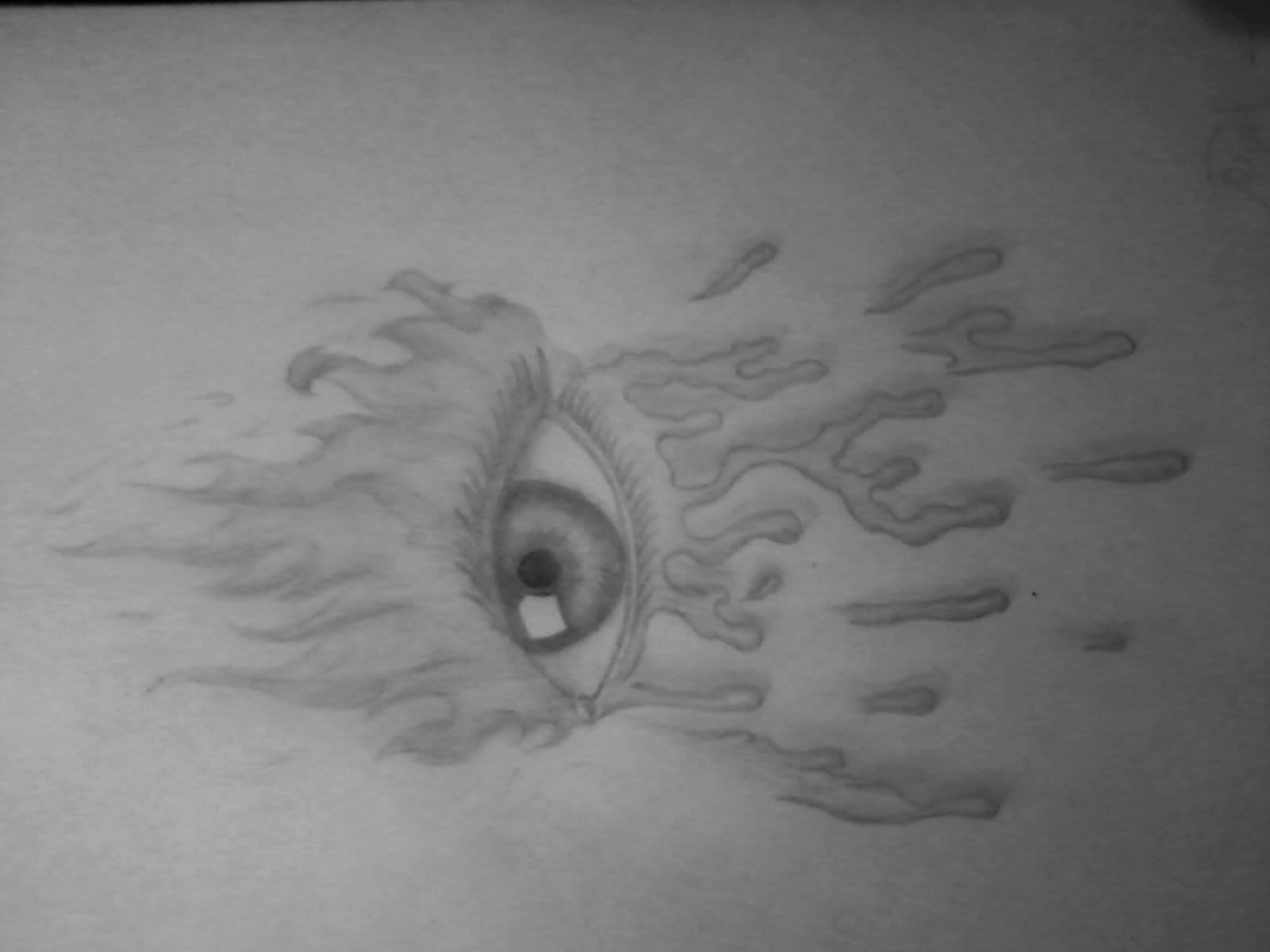A detailed, cleaned-up caption for the described image could be:

"This pencil-drawn illustration features a detailed eye rendered in grayscale tones. The eye, oriented sideways, showcases meticulously drawn eyelashes and a prominently shaded iris and pupil. A reflective highlight adds a touch of realism to the pupil. Surrounding the eye, a dynamic, fiery pattern emanates from above (or from the left, given the eye's orientation), while beneath the eye, a depiction of water droplets appears to cascade downwards. The entire artwork is set against a white background, emphasizing the contrast and texture provided by the pencil shading."